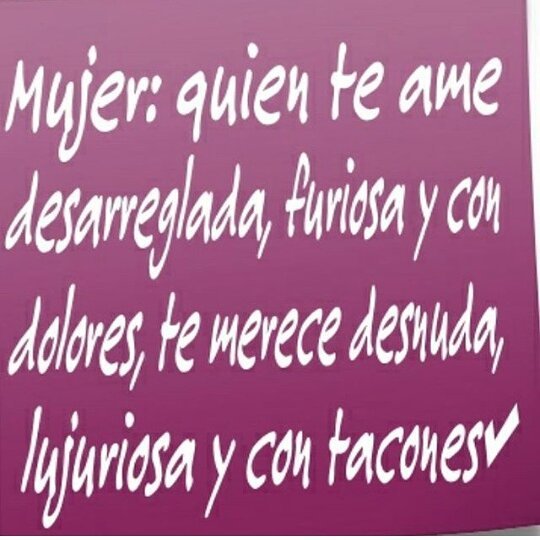The image depicts a poster board written in a foreign language, possibly Arabic or another Middle Eastern language. The text is emblazoned in white letters on a predominantly fuchsia, or burgundy background. The lettering spans from the top left corner and continues downwards. Notably, in the lower right-hand corner, there is a distinct white check mark. The poster presumably acts as an advertisement and occupies the entire frame of the photograph, suggesting it might be situated in a public space, such as a street or restaurant.